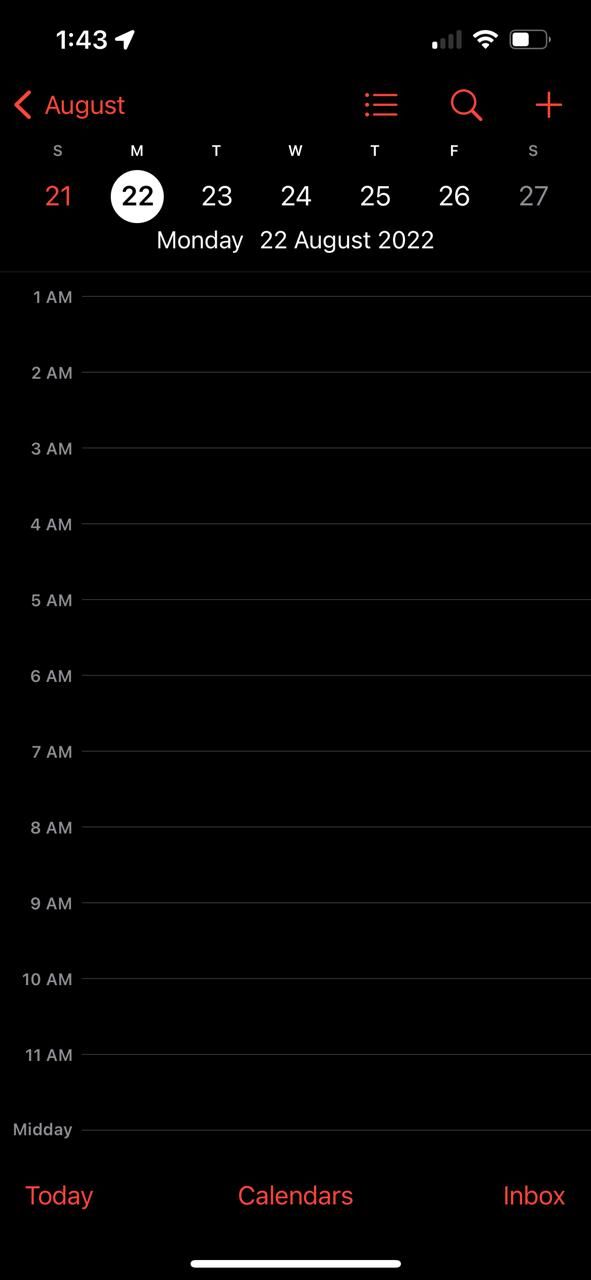A screenshot captured from a mobile device displays a detailed view of a calendar app. The top of the screen features white status icons indicating the time, network connection, Wi-Fi connectivity, and battery life. The background of the screenshot is black, with text displayed in white and red for contrast. The calendar is set to Monday, 22nd August 2022, and the day's schedule is segmented into hourly intervals, starting from 1 AM and extending to midday, each hour divided by thin white lines. 

At the bottom of the screen, there are three navigation options labeled "Today," "Calendars," and "Inbox." The top of the screen includes a red magnifying glass icon for search, a cross icon for close or delete functions, and an icon consisting of bullet points with three horizontal lines, presumably representing menu options or additional settings.